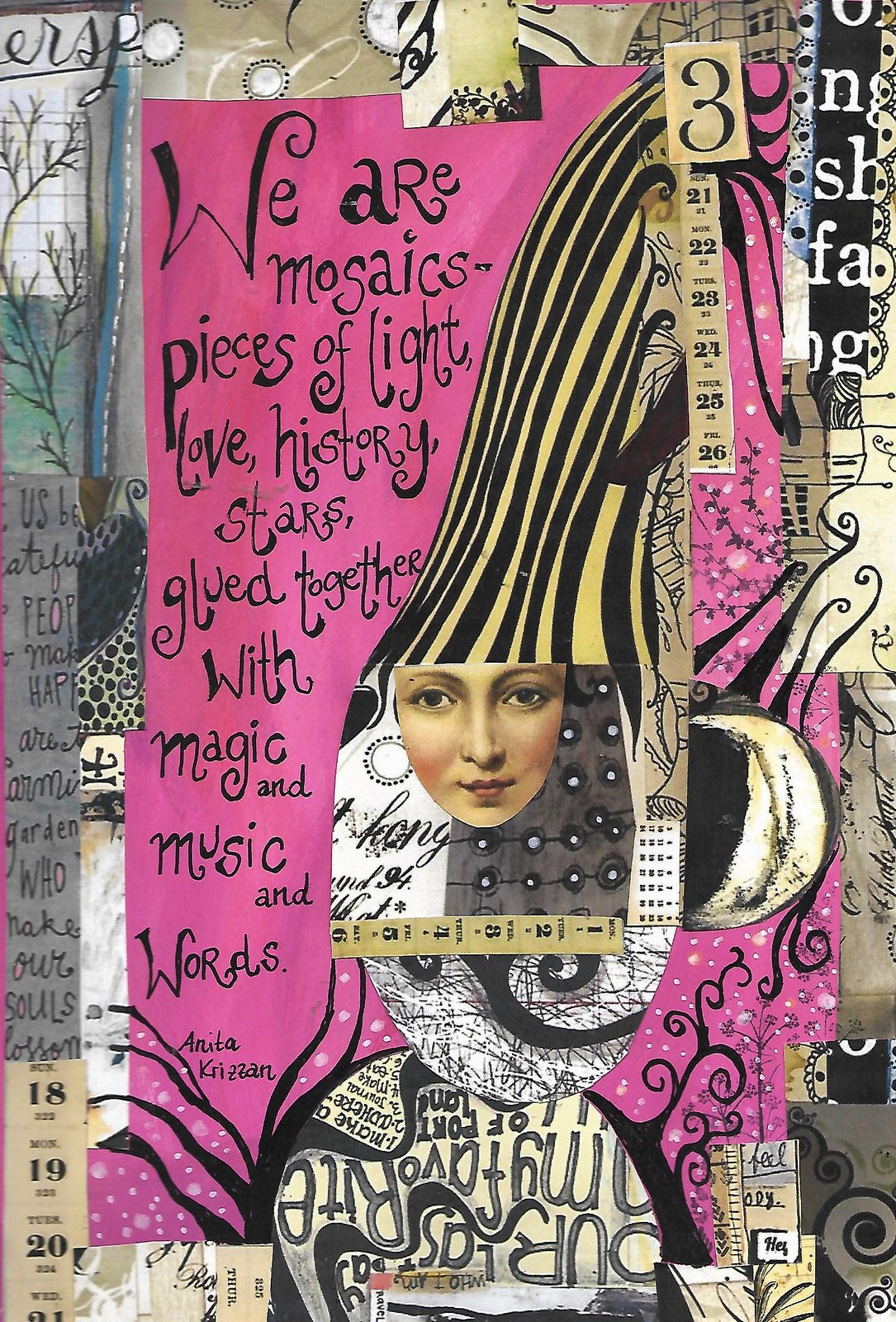This image showcases a heavily detailed artistic collage with a predominantly pink theme. Central to the artwork is a painting of a woman's face adorned with prominent blush and red lipstick. Her visage is complemented by strands of gold and black, suggestive of her hair. To the left, there's a painting featuring a leafless tree. Dominating the collage is a poetic quote handwritten in a fancy, artistic style that reads: "We are mosaics, pieces of light, love, history, stars, glued together with magic and music and words." This quote is attributed to Anita Krizzan. The collage also includes various elements such as strips of paper with the numbers 18, 19, 20, 21, and multiple design elements like dots, circles, and letters. Additionally, there are sections of grey, black, blue, and beige interspersed within the artwork, providing a subtle contrast to the pervasive pink hues.